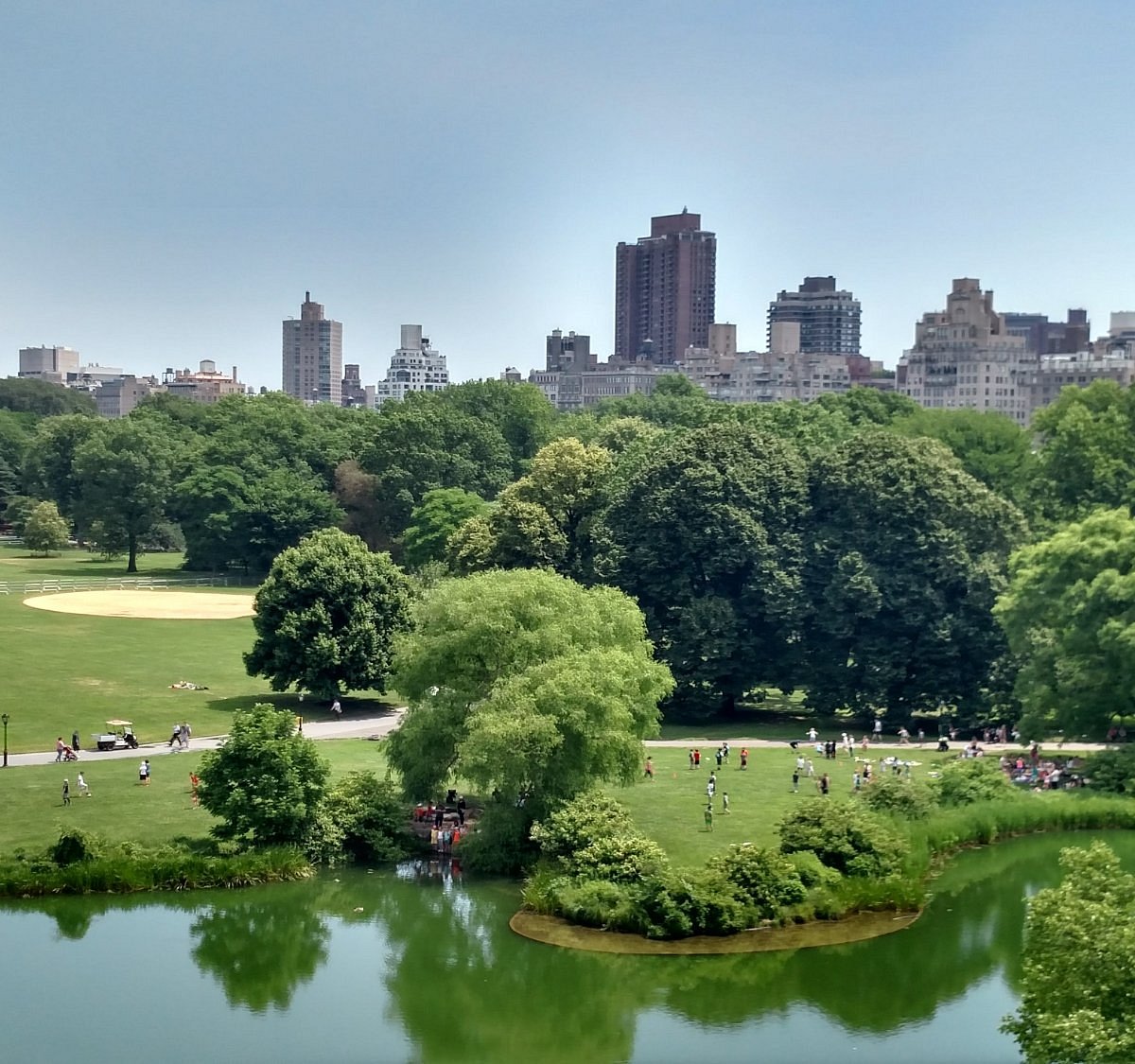The photograph showcases a vibrant outdoor scene on a sunny day, capturing the serene beauty of nature intertwined with urban life. At the bottom of the image, a small pond lies with its greenish water reflecting the lush trees and shrubs along its shore. The water's green hue is likely due to these reflections. Beyond the pond, numerous people gather in a grassy area, some enjoying picnics towards the right. A walkway or street cuts through this lively setting, with a golf cart visible on the far left, suggesting the presence of a golf course. To the left of the image, a fenced sand pit, likely a sand trap, complements the golf course theme. Dense trees with various shades of green leaves frame the background, creating a verdant tapestry. Above these trees, a sprawling cityscape emerges, featuring an array of medium to tall high-rise buildings, predominantly on the right, with some appearing further away on the left. The sky above is a clear, bright blue, encapsulating the essence of a perfect midday.